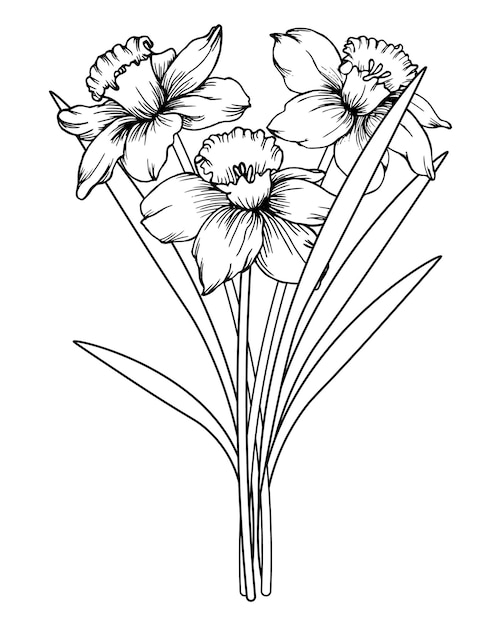This image exhibits a detailed black and white pen drawing of three daffodils set against a plain white background. The flowers have long, slender stems that converge at the base of the drawing, which measures approximately four inches in height and up to four inches in width at its broadest point. Each daffodil features prominently with a raised bell-shaped center displaying delicate stamens, surrounded by six pointed, wide petals, indicating they are in full bloom. There are four elongated, bunny ear-like leaves, each about a quarter of an inch wide, the longest extending up to four inches in length, flanking the stems on both sides. The combined effect is an elegant and somewhat delicate illustration with thick, defined outlines that give it an intricate, yet simplistic beauty, highlighting the symmetry and natural grace of the daffodil flowers.